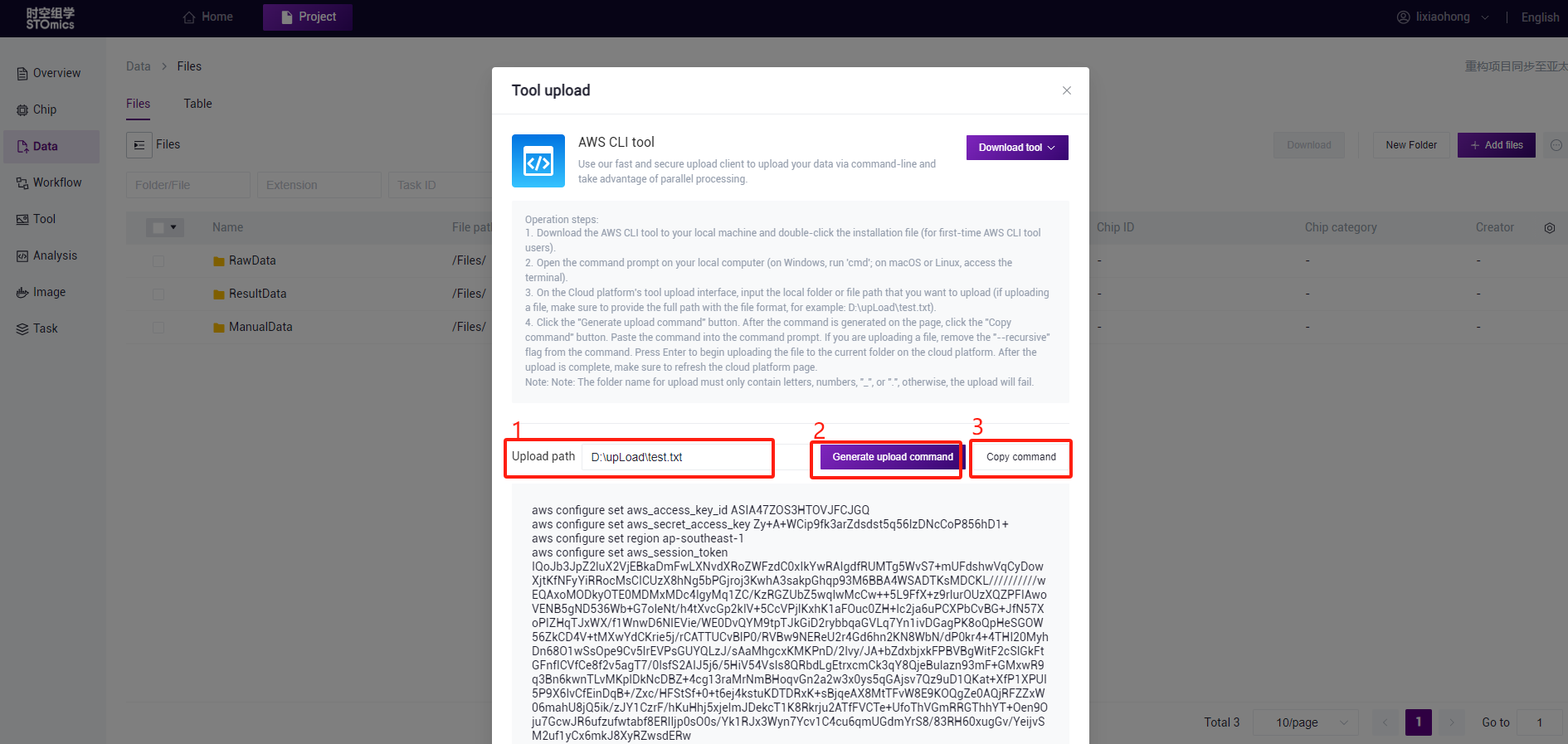### Detailed Caption for Website Screenshot:

This is a detailed screenshot capturing a segment of a website focused on tool upload functionalities. The image has a layered composition, with the website's main interface appearing small and slightly grayed out in the background, while the forefront is in sharp focus with a bright white background. 

On the left-hand side, partially visible categories listed in the grayed-out menu include "Overview," "Chip," "Data," "Workflow," "Tool," "Analysis," "Image," and "Task." These categories hint at the website's multifaceted nature, likely geared towards data management or a technical workflow.

Dominating the brighter forefront of the screenshot is the "Tool Upload" section. Here, the text "AWS CLI Tool" is prominently displayed next to a distinctive blue icon, suggesting the tool involved is related to Amazon Web Services' Command Line Interface. Adjacent to this, on the right, is a "Download Tool" button highlighted in purple, indicating an action item for users.

Key elements in the middle of the screen are emphasized with red highlights and enumerated labels:
1. **Upload Path:** Displayed with a designation of "Drive D," this is marked by a red rectangle, indicating where users should specify the upload path.
2. **Button (Text Unclear):** A second red-highlighted item, noted as a purple button, is present but its tiny text is unreadable in the screenshot.
3. **Copy Command:** The third highlighted area, also enclosed in a red rectangle, includes a "Copy Command" prompt, suggesting a quick way to copy necessary command lines.

Overall, this screenshot appears to be a part of a how-to guide, aiding users in uploading tools to a specified platform. Despite the background content being mostly unreadable due to its small size, the clear emphasis on certain interactive elements brings attention to critical steps in the upload process.